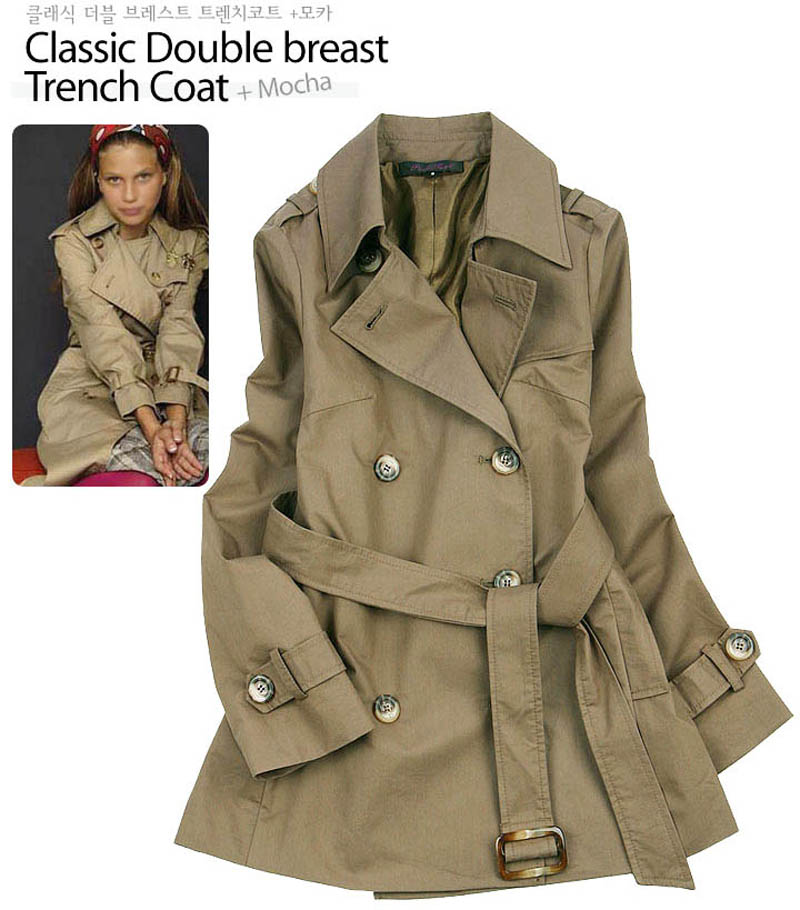This photograph serves as an advertisement for a "classic double-breast trench coat," featuring a light brown or beige trench coat prominently displayed against a white background. The coat showcases seven visible buttons, which are silver or gray, and is complemented by a golden or brown belt buckle. Additionally, the coat has long sleeves with loops and thick beige collars, plus a visible inner tag. 

In the upper left corner of the image, there is black text that reads "classic double breast trench coat plus mocha," with Chinese lettering above it. Nearby, there is an inset photograph of a young woman with straight brown hair, wearing a red and white headband, sitting on a red platform. She wears the same trench coat over a dress and gazes at the camera with a slight smile. Her arms are extended, adding a dynamic element to the composition.